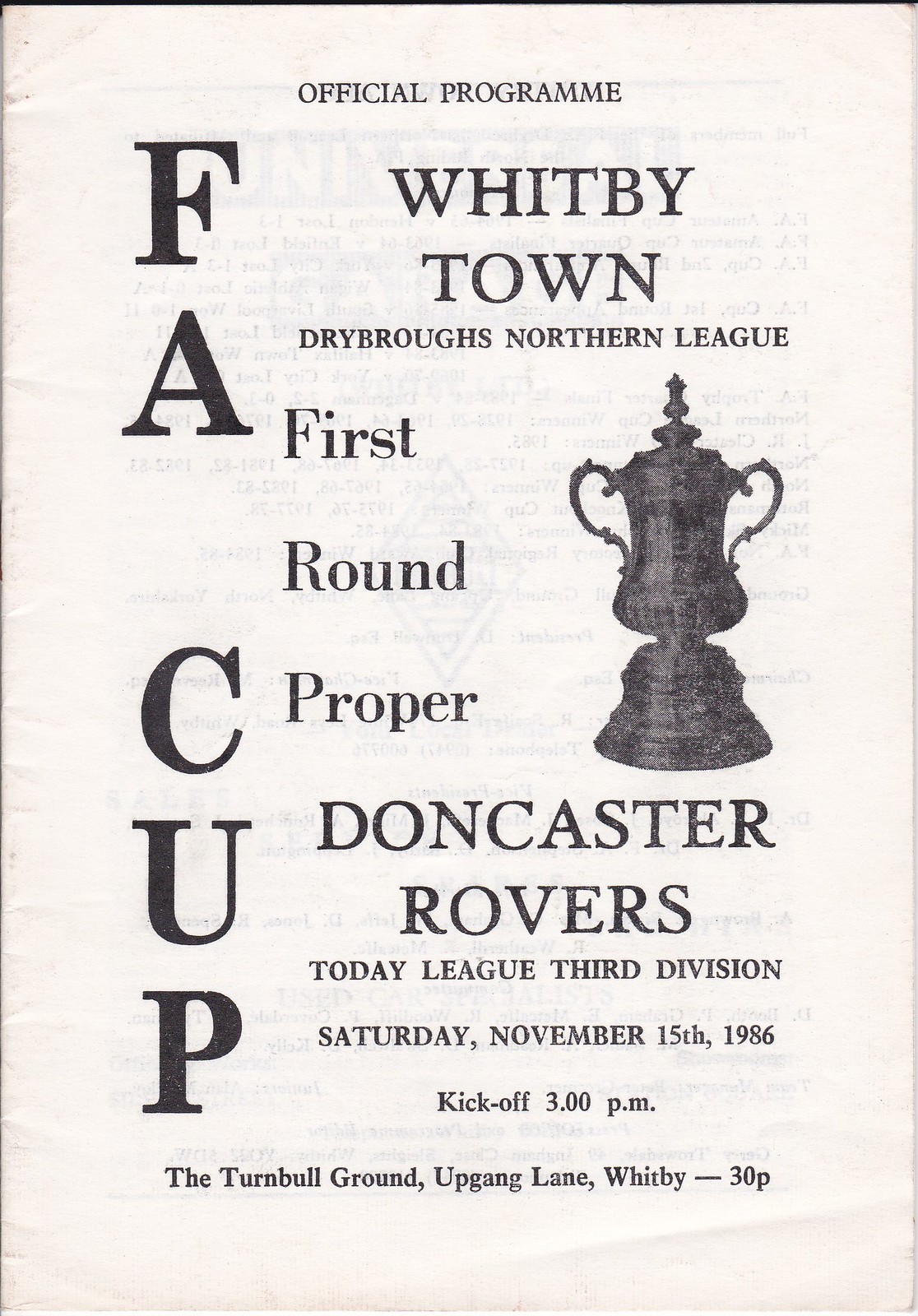The image is a cover for an official soccer program, featuring a minimalistic white background with bold black text. The text on the cover reads as follows: "Official Program, Whitby Town vs. Dry Boroughs, Northern League, First Round Proper, Doncaster Rovers, Today League, 3rd Division. Saturday, November 15th, 1986. Kickoff, 3pm. The Turnbull Ground, Upgang Lane, Whitby, 30P." 

Running vertically along the left side of the cover is the text "F.A. Cup," and to the right is an outline of a black trophy cup. The trophy cup is designed as a chalice with a round base, topped with a small knob for a lid, and features two handles. The overall aesthetic is black and white, with the white paper showing subtle signs of wear, including some text from the next page faintly visible through it.